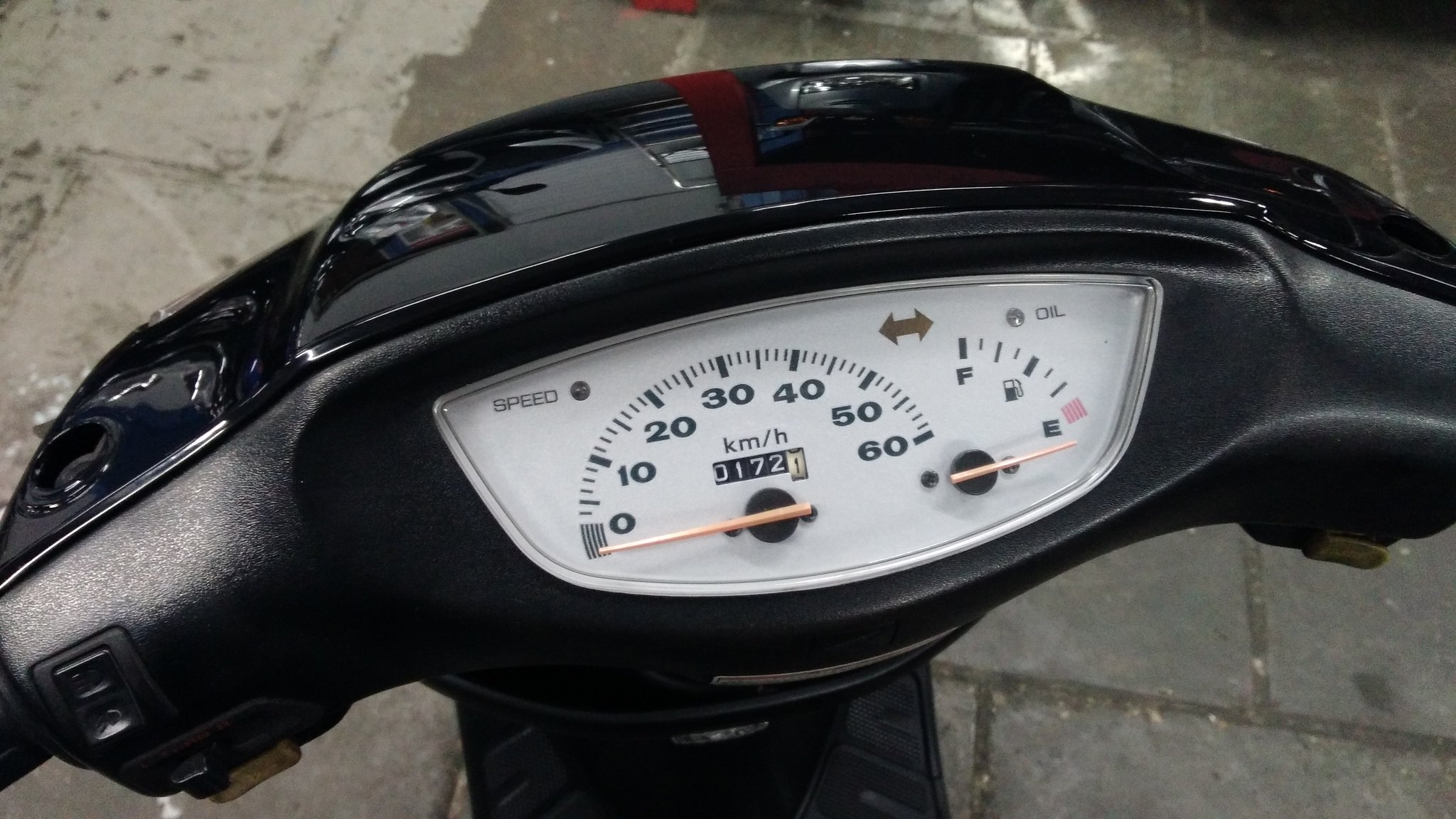The image displays a close-up, first-person view of a moped's handlebars and speedometer. The moped, predominantly black, is centrally positioned within the frame. The white-faced speedometer features black text, with "SPEED" indicated on the left and "OIL" on the right, and includes a fuel gauge that appears to show empty, likely due to the moped being turned off. The speedometer measures in kilometers per hour, ranging from 0 to 60. The scene is set on a gray-tiled surface, suggestive of a back patio or a sidewalk, providing a neutral, even-toned background that contrasts with the moped's dark color.